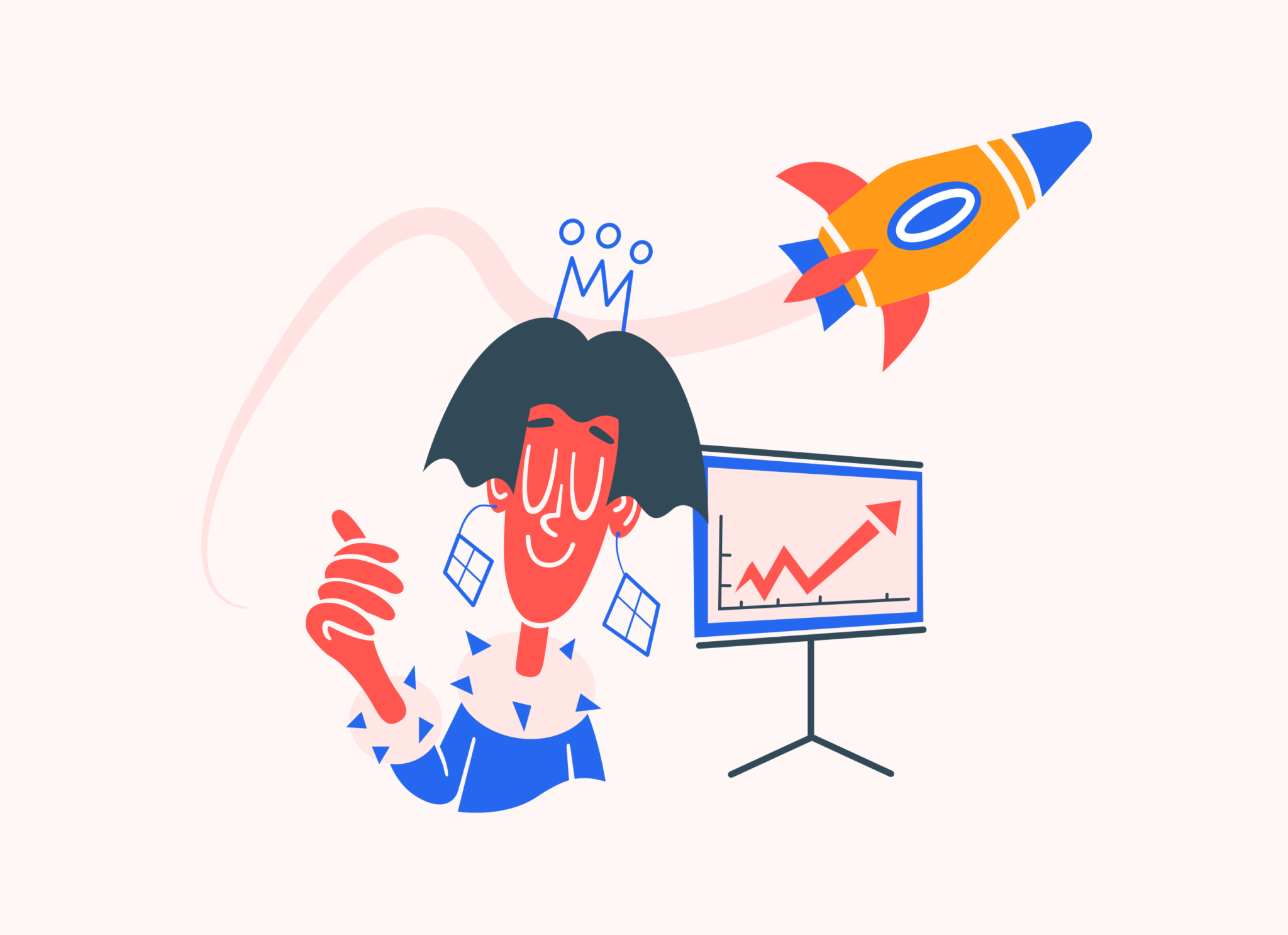The image depicts a cartoonish vector graphic of a monarch figure, likely a queen, characterized by bright colors and a distinctive art style reminiscent of Corporate Memphis. The queen features short, nearly black hair, closed smiling eyes shaped like U's, and a stylized nose and white mouth. Her orange-hued skin contrasts with her blue outfit, which includes a dress and cuffs adorned with small blue triangles. She wears a thin, three-pointed blue crown topped with small circles and blue, window-logo-like earrings.

In the background, a light pink hue sets the scene, with two notable elements: an orange rocket ship with blue accents, including its nose, window, and rear engine section, ascending from the top of the image, and a chart on the bottom right corner displaying a red arrow pointing upwards, suggesting financial growth or stock market trends. The overall setting is bright with clear visibility, indicating a polished and intentional design likely used for presentations on investment or financial topics.